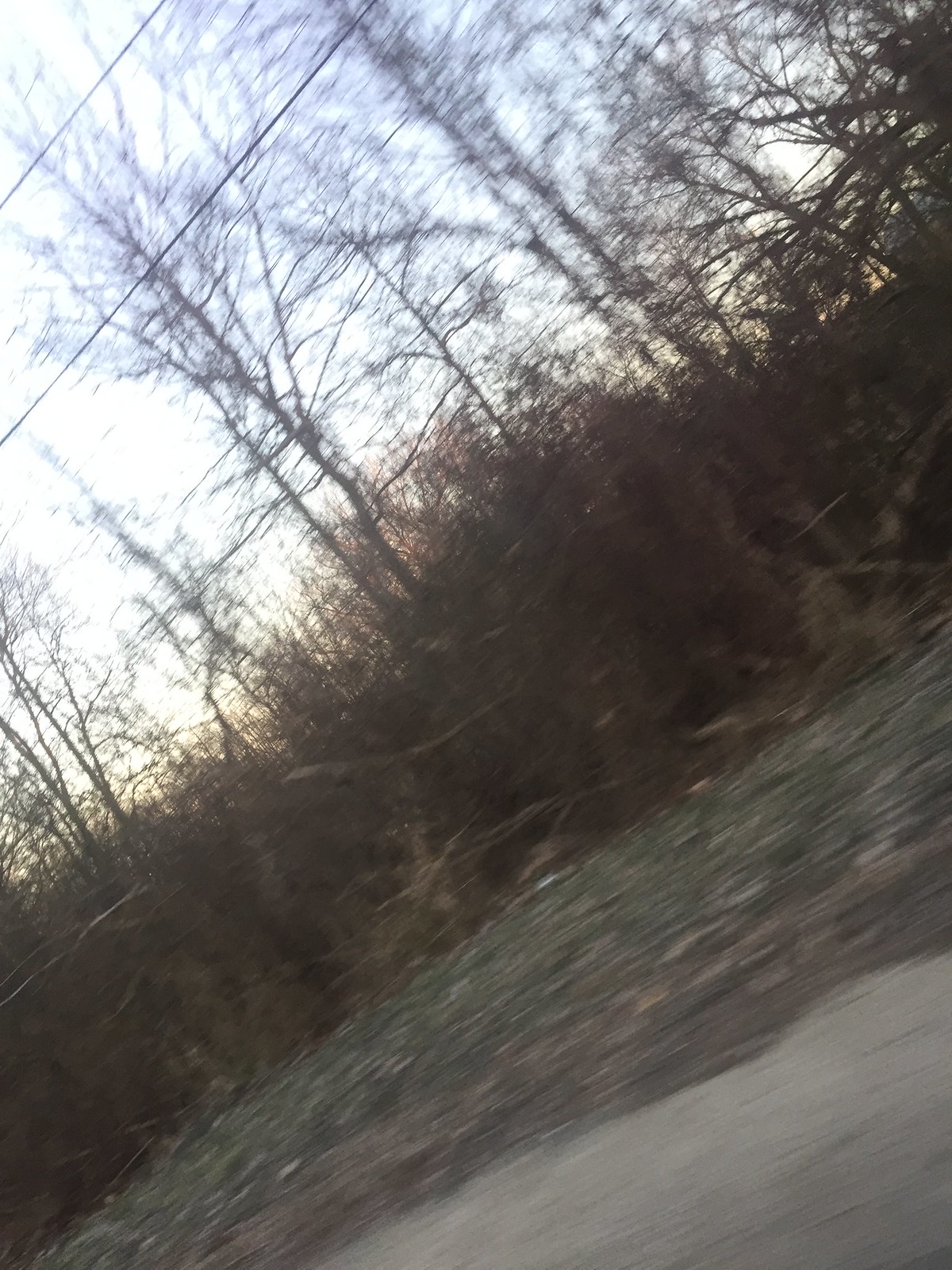The image depicts a blurry, grainy photograph likely taken from a moving vehicle, capturing an outdoor scene at either dusk or very early in the morning. The lighting is poor, contributing to the overall low quality and various shades of brown throughout the picture. The scene includes a small section of road and a sandy pathway at the bottom, leading to rough ground scattered with stones and patches of dark green and yellowish grass. A variety of trees dominate the background, ranging from tall, thin, leafless trees to shorter, bushier shrubs, all appearing barren, suggesting it was taken in the fall or winter. Overhead, faint power lines are visible, adding to the impression of a roadside setting. The entire scene feels somewhat dismal and lifeless, enveloped in shadowy light just before nightfall.